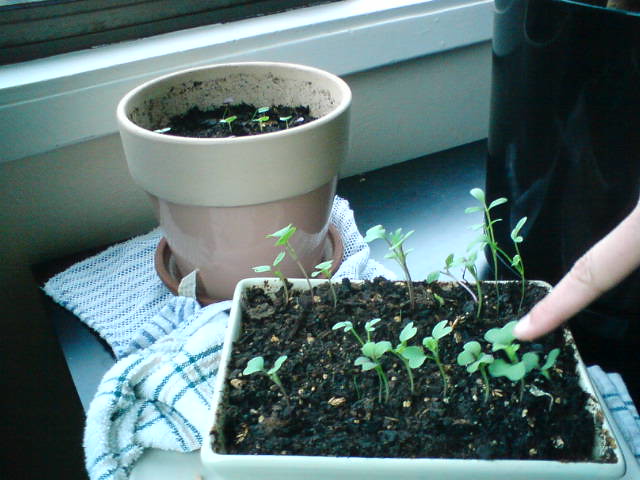The photograph shows a close-up of a windowsill area with a white window trim in the upper left-hand corner and a white wall extending below. The image is taken from a diagonal perspective, revealing two distinct pots containing small green seedlings. A rectangular pot filled with dark soil and sparse, small green plants sits on a striped black, blue, and white cloth. To the right, a round light brown pot with similar contents rests on a different cloth featuring a plaid design of blue, white, and gray. A light-colored finger on the right-hand side points towards the seedlings in the rectangular pot, emphasizing their tiny green leaves sprouting from the soil. The background includes a table or counter surface covered by the cloths. Additionally, the upper right-hand corner of the photograph shows a shiny black object partially cut off. The overall scene is illuminated by light coming from the windowsill, casting a natural glow over the setup.